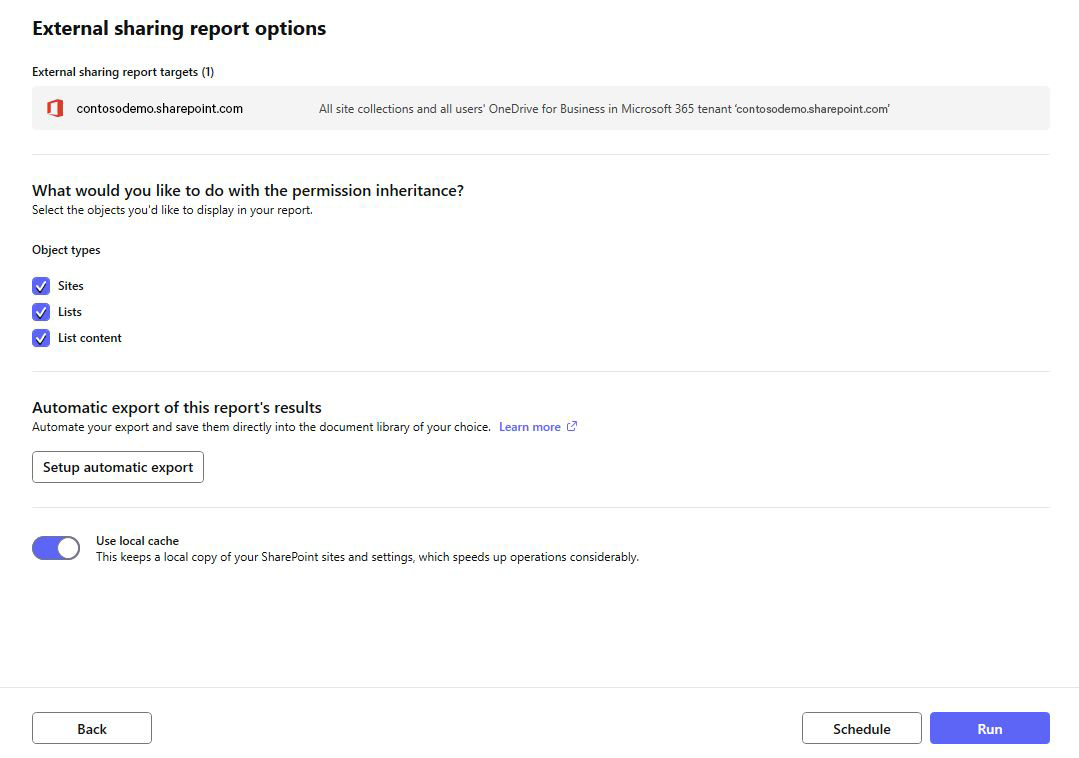The image is a detailed interface for configuring external sharing reports from a SharePoint site. At the top, bold text reads "Top External Sharing Reports Options," followed by smaller text specifying "External Sharing Report Targets (1)." Below this, an icon featuring a squared shape precedes the text "CONTOSODEMO.SHAREPOINT.COM." The description continues, stating that all site collections, all users, OneDrive for Business, and Microsoft 365 within the tenant "CONTOSODEMO.SHAREPOINT.COM" are included.

A light gray line separates this section from the next, where bold text asks, "What Would You Like to Do with Permission Inheritance?" This is followed by instructions to "Select Objects You Would Like to Display More in Your Report," with options for "Sites," "Lists," and "List Content," each accompanied by a blue check mark on the left.

Another section in bold mentions "Automatic Export of This Report's Results," with additional details stating, "Automate Your Report and Save Them Directly into the Document Library of Your Choice," followed by a "Learn More" link marked with an upper-right-hand arrow. Within a black box, the text "Setup Automatic Export" appears prominently.

Next, a toggle button labeled "Use Local Cache" is depicted as clicked to the right. This option explains that it "Keeps a Local Copy of Your SharePoint Sites and Settings, Which Speeds Up Operations Considerably."

At the bottom, there are two separate rectangle boxes outlined in black, each containing bold text—one says "Back" and the other "Schedule."